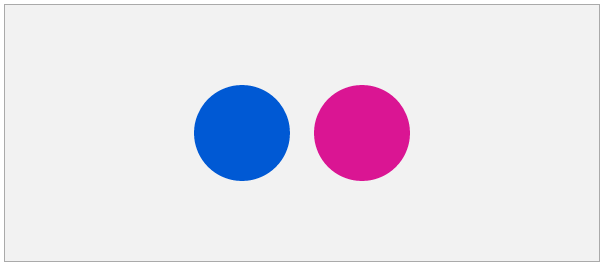The image features a minimalist design with a plain background that is a subtle mix of white and light gray. At the center of this clean background are two identically-sized circles placed side-by-side. The circle on the left is a vibrant indigo, resembling the color of an indigo balloon. Adjacent to it on the right is another circle, filled with a striking fuchsia hue. Both circles are smooth and seamless, with no visible outlines, emphasizing their bold colors against the understated backdrop.